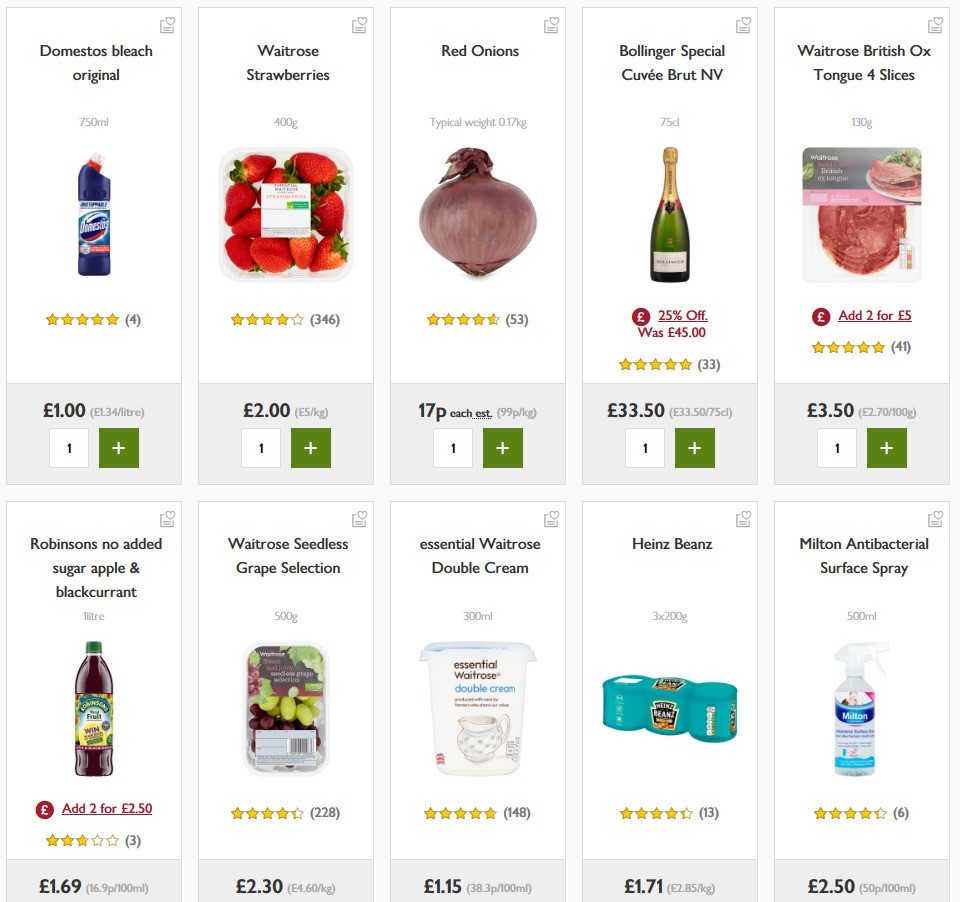This screenshot displays a selection of items available for purchase, presented against a white background. In the first row, from left to right:

1. The first item is "Domestos Bleach Original," priced at £1. The corresponding image of the Domestos bleach bottle is shown.
2. To the right, there is a package of "Waitrose Strawberries," with a four-star rating out of five based on 346 reviews, and priced at £2. An image of fresh strawberries is shown.
3. Below the strawberries, there is an image of a fruit drink. The caption reads "Add two for £2.50." The drink has a three-star rating out of five from three reviews and is priced at £1.69.
4. To the right of the fruit drink, there is a package of mixed red and green grapes. This item has received 228 reviews, gaining a four-star rating, and is priced at £2.30. An image of the grape package is included.